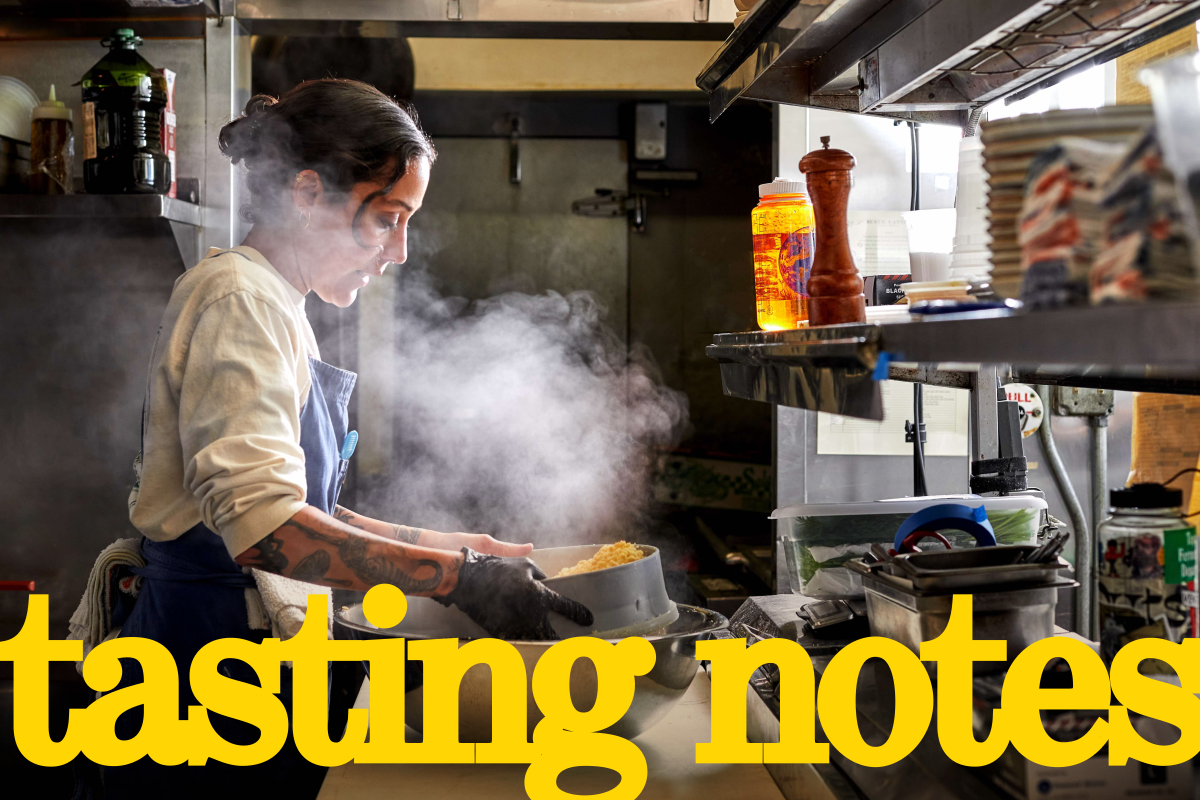In this image, a young woman with dark, tattooed arms is preparing food in a professional kitchen. She’s wearing a white shirt with sleeves rolled up, a blue apron, and a black glove on her right hand. Her hair is pulled back into a bun. She is focused on mixing noodles that are steaming in a bowl in front of her, and she has a towel tucked into her back pocket. The kitchen around her is equipped with various utensils and ingredients; a brown pepper mill, stainless steel trays, canisters, and a water bottle are visible. Shelves stocked with equipment and a large stainless steel cooler, possibly a walk-in, can be seen in the background. The photo features big, bold yellow lettering at the bottom reading "Tasting Notes." The scene captures the essence of culinary preparation and the meticulous environment of the kitchen.